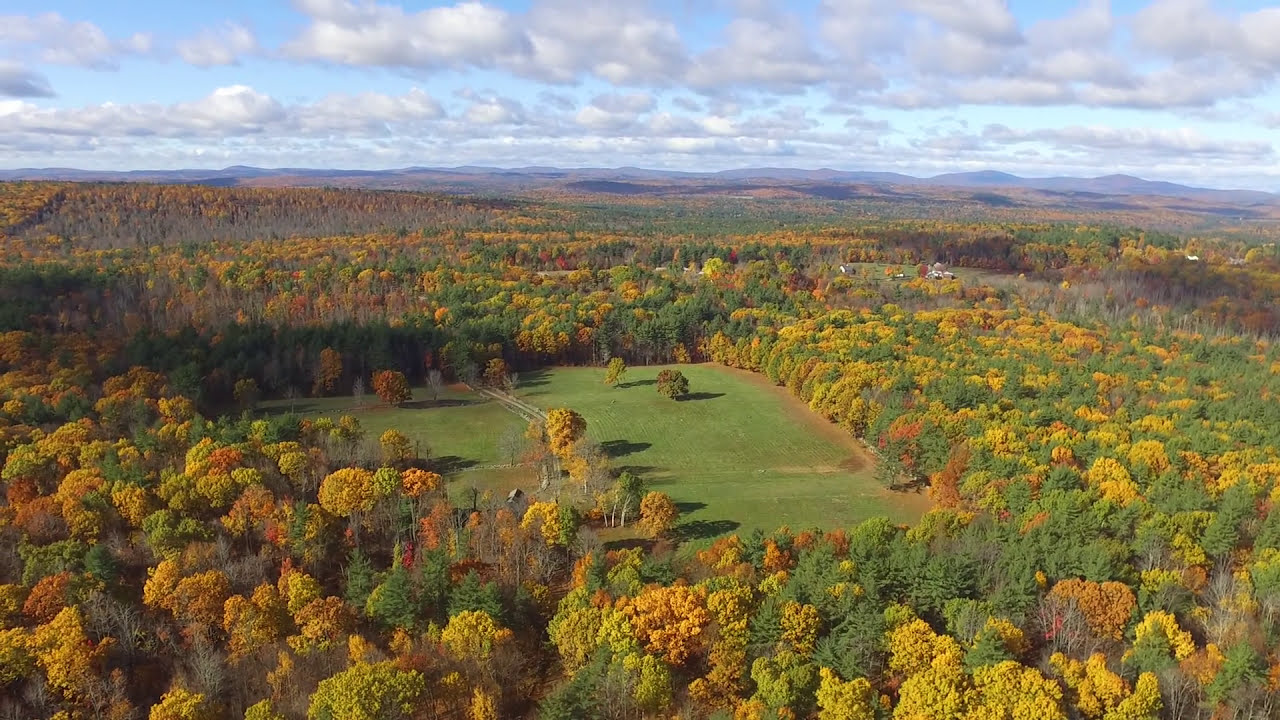The image is a breathtaking aerial photograph capturing a picturesque countryside in the midst of autumn. The trees are painted in a stunning palette of green, yellow, brown, orange, and red, signaling the fall season. Nestled among these vibrant autumnal trees, a lush green field lies center-left, crossed by a small path, with a couple of scattered trees dotting its expanse. In the foreground, a small building peeks through the tree line, revealing the presence of a quaint village or small town nearby. As the landscape stretches out, it transitions into rolling hills and, in the far distance, majestic mountains rise under a bright blue sky adorned with several fluffy, white clouds. The sunlight filters through, casting reflections on the distant mountains, adding to the idyllic and serene atmosphere of this captivating scene.